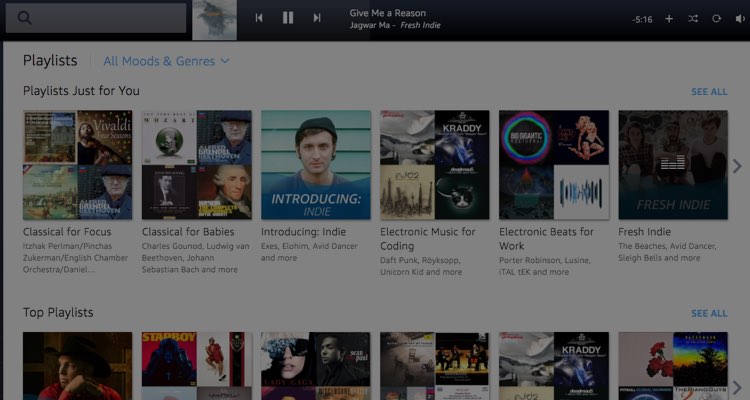The image showcases a YouTube playlist interface with a currently playing video at the top titled "Give Me a Reason by Jaguar Ma" from the album "Fresh Indie." The exact moment captured obscures the video thumbnail, but the title is clearly visible. Below the video, against a white background, there is black text in the top left reading "Playlists," and to the right, light blue text displays "All Moods and Genres." Further down, in black text, it says "Playlists Just for You," followed by a horizontal row of curated playlist suggestions. These include "Classical for Focus," "Classical for Babies," "Introducing Indie," "Electronic Music for Coding," "Electronic Beats for," and "Fresh Indie," each accompanied by its own thumbnail image. Additionally, there's a second horizontal list of top playlists, but the image is cut off midway through this section, so not all thumbnails are visible.